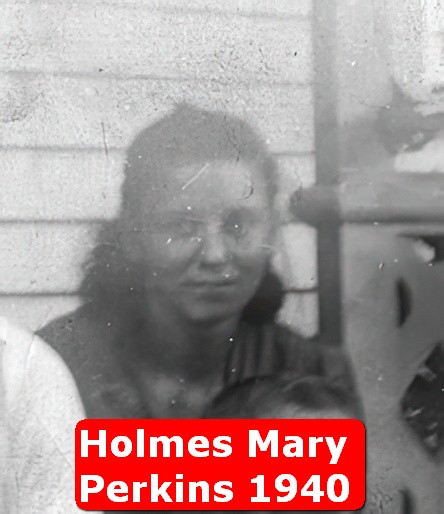This image is a worn and scratched black and white photograph with shades of red, white, black, and various grays. The old and weathered photo depicts a woman with brunette or dark hair positioned directly in the center, gazing slightly off to the side towards the camera. The background suggests an outdoor setting, possibly in the middle of the day. On the right side of the image, there's a door visible, and at the bottom left, an individual is partially cut off. At the bottom of the image, there's a distinct red rectangle with rounded corners containing white text that reads, "Holmes, Mary Perkins, 1940."